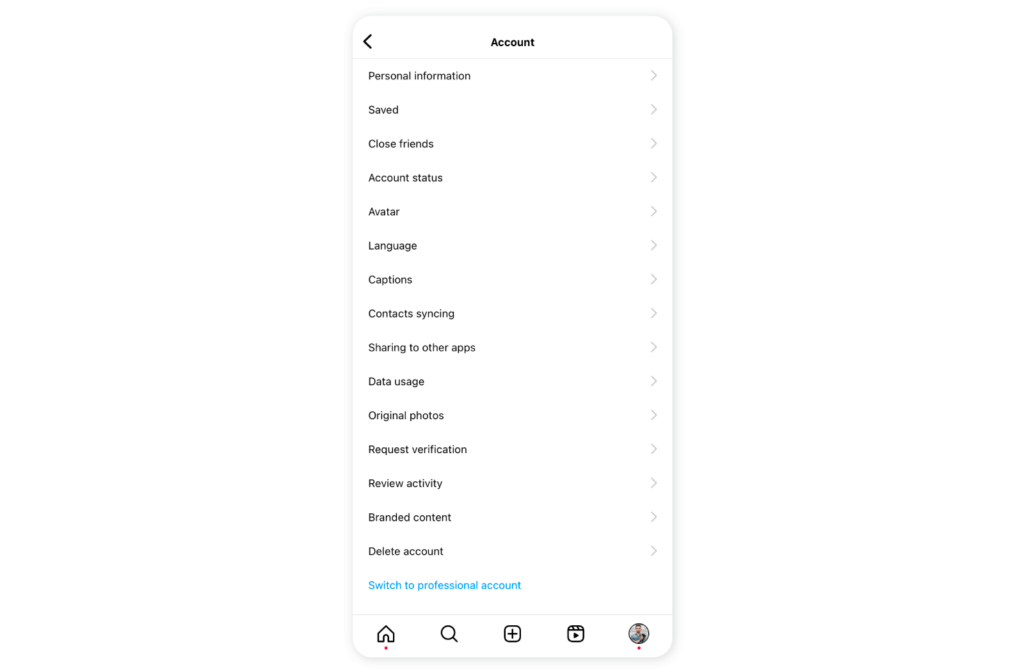This image showcases a smartphone screen with a user interface designed for account settings. The screen features a white background, black text, and gray outlines along the edges. At the top, a black arrow pointing to the left is followed by the word "Account" in the center. Below this, a gray line spans horizontally.

Each subsequent line on the interface lists a different setting, each accompanied by a gray arrow on the right:

- **Personal Information** followed by a gray arrow.
- **Saved** followed by a gray arrow.
- **Close Friends** followed by a gray arrow.
- **Account Status** followed by a gray arrow.
- **Avatar** followed by a gray arrow.
- **Language** followed by a gray arrow.
- **Captions** followed by a gray arrow.
- **Contact Syncing** followed by a gray arrow.
- **Sharing to Other Apps** followed by a gray arrow.
- **Data Usage** followed by a gray arrow.
- **Original Photos** followed by a gray arrow.
- **Request Verification** followed by a gray arrow.
- **Review Activity** followed by a gray arrow.
- **Branded Content** followed by a gray arrow.
- **Delete Account** followed by a gray arrow.

Below these settings, a blue font indicates the option to **Switch to Professional Account**, with another gray line beneath it.

At the bottom of the screen, five icons are positioned from left to right:

- A gray outlined house with a red dot underneath.
- A gray magnifying glass indicating the search button.
- A rounded square with a black cross in the middle.
- Another rounded square with a black triangle pointing to the right.
- A circle featuring an image of a person with a red dot underneath.

This detailed layout provides a comprehensive view of the account settings interface on the device.